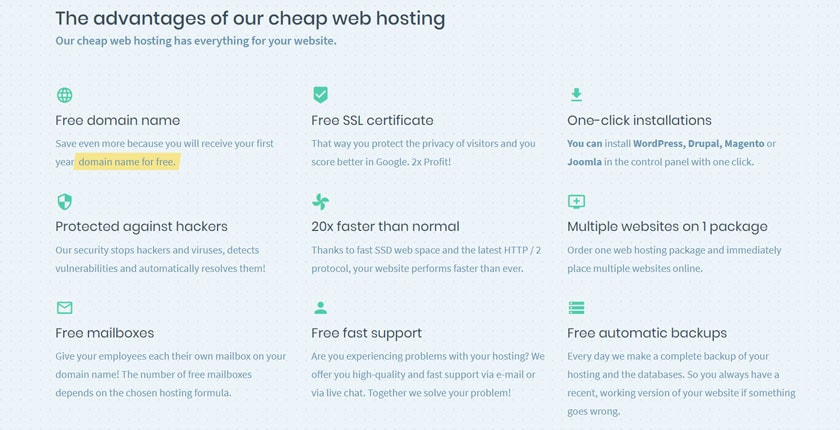This image is a cropped screenshot highlighting the benefits of a web hosting platform. The image has a light blue background with a subtle dotted texture. At the top of the image is a heading in rounded, almost geometric sans-serif letters that states, "The Advantages of Our Cheap Web Hosting." The color of the text appears to be either black or dark blue. Just below the heading, there is a subheading in light blue text that reads, "Our cheap web hosting has everything for your website."

The content is organized into three columns, each containing three sections, making a total of nine sections. Each section includes an icon, a heading, and a paragraph of descriptive text.

- **Column One:**
  1. **Free Domain Name:** Includes a green earth icon. The subtext reads, "Save even more because you will receive your first domain name for free," with "domain name for free" highlighted in yellow.
  2. **Protected Against Hackers:** Features a shield icon. The subtext indicates, "Our security stops hackers and viruses, detects vulnerabilities, and automatically resolves them."
  3. **Free Mailboxes:** Represented by a mail icon, accompanied by relevant information about the mail service.

- **Column Two:**
  1. **Free SSL Certificate:** Depicted with a green banner icon with a white checkmark. The subtext provides additional details.
  2. **20x Faster than Normal:** Illustrated with a fan icon. The subtext explains the speed benefits.
  3. **Further Features:** Continues with additional benefits presented in a similar structured format.

- **Column Three:**
  1. **(Details of the feature in the first section of the third column)**
  2. **(Details of the feature in the second section of the third column)**
  3. **(Details of the feature in the third section of the third column)**

This visually engaging layout is designed to clearly present the various advantages of the web hosting service, making it easy for users to quickly grasp the key features offered.